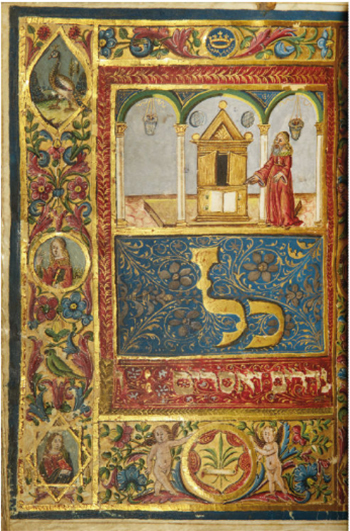This highly detailed, medieval-style artwork combines rich colors and intricate patterns, enclosed within multiple borders: a beige outer border, followed by a dark navy one, and an inner greenish border accented with floral prints. The artwork's central theme appears to focus on a man in a red robe standing beside a small golden building, possibly under an archway. Above, a blue section showcases floral designs and two vertical golden lines, while below, a red section contains gold lettering. The bottom of the piece features two naked cherubs or babies around a gold circle containing a red, green, and gold crest or shield. On the left, there are more figures and floral patterns, and the presence of ducks and peacocks adds a touch of whimsy. The piece could be a quilt, a painting, a medieval manuscript page, or even a decorative fabric, underscoring its enigmatic origin and historical charm.